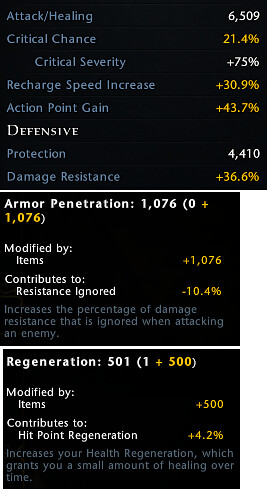The image is a set of three text boxes arranged in a landscape orientation against a black background, depicting detailed statistical information from a video game. The top box, which is slightly wider than the two below it, lists various player stats in blue and white typography with some score tallies in yellow. The categories include Attack/Healing (6,509), Critical Chance (21.4%), Critical Severity (+75%), Recharge Speed Increase (+30.9%), Action Point Gain (43.7%), Defensive Protection (4,410), and Damage Resistance (+36.6%). The second box focuses on Armor Penetration, with details modified by items and contributing to resistance ignored. The third box details Regeneration (501), noting modifications by items and contributions to hit point regeneration. The overall design combines color typography and graphic design elements to present comprehensive statistical information.